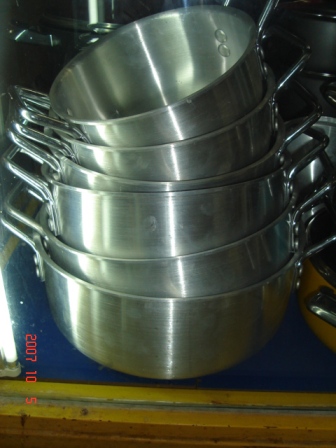A small, color photograph dated 2007-10-5, taken in portrait format, features a stack of six stainless steel saucepans nestled inside each other like Russian nesting dolls. The date stamp, in orange text, is located in the lower left corner and can be read vertically when the image is rotated 90 degrees clockwise. The pans are positioned slightly crooked and tipping to different sides, with dual handles riveted on both the left and right. They rest on a yellowish wooden surface that appears to be a kitchen counter, topped with a dark blue mat or placemat. A vertical white tube light to the left of the image casts illumination, creating shadows and reflections that form two distinct lines up the side of the stacked pans—a wider line on the left and a narrower one near the center. The overall image is dark around the edges, emphasizing the central arrangement of the cookware.